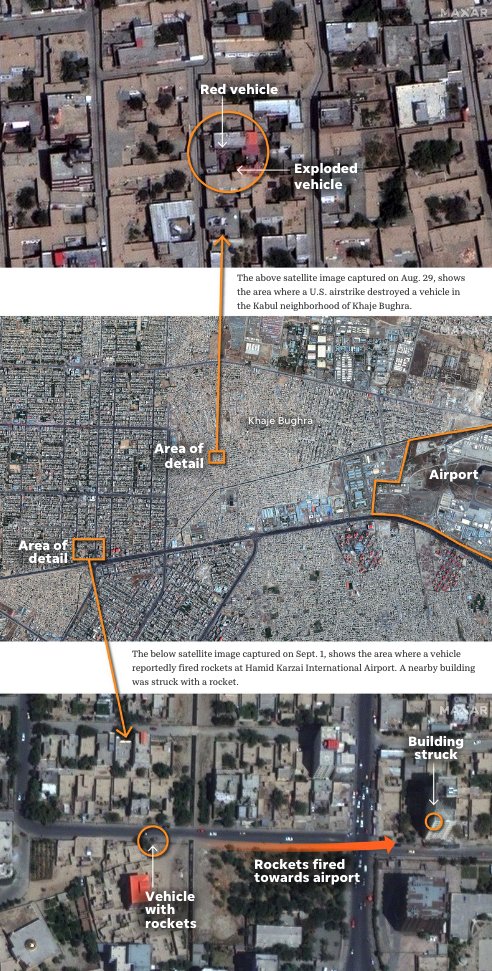This composite aerial image consists of three photographs aligned vertically, each detailing different aspects of a cityscape related to significant events. The top image provides an overhead view of a Kabul neighborhood, specifically highlighting the aftermath of a U.S. airstrike on August 29th. This image marks a red vehicle circled in yellow, with a white arrow and label pointing out an exploded vehicle nearby.

The middle image displays a broader, satellite perspective of the area, labeled "Khaji Bughra." Key annotations include a yellow square referencing the detailed area in the top image and directional markers towards the Hamid Karzai International Airport. This section provides geographic context and shows more extensive urban surroundings with smaller, less distinct objects.

The bottom image, another detailed aerial shot, is zoomed in similarly to the top image but focuses on a different event. Captured on September 1st, it highlights a vehicle with rockets presumably used to fire at the airport. Important markings include a circle around the rocket-laden vehicle, an arrow indicating the direction of the fired rockets, and a yellow circle highlighting a building struck by one of the rockets.

Together, these images track and provide detailed evidence concerning hostile activities in the city, with clear visual distinctions and annotations to aid in understanding the sequence and impact of the incidents.